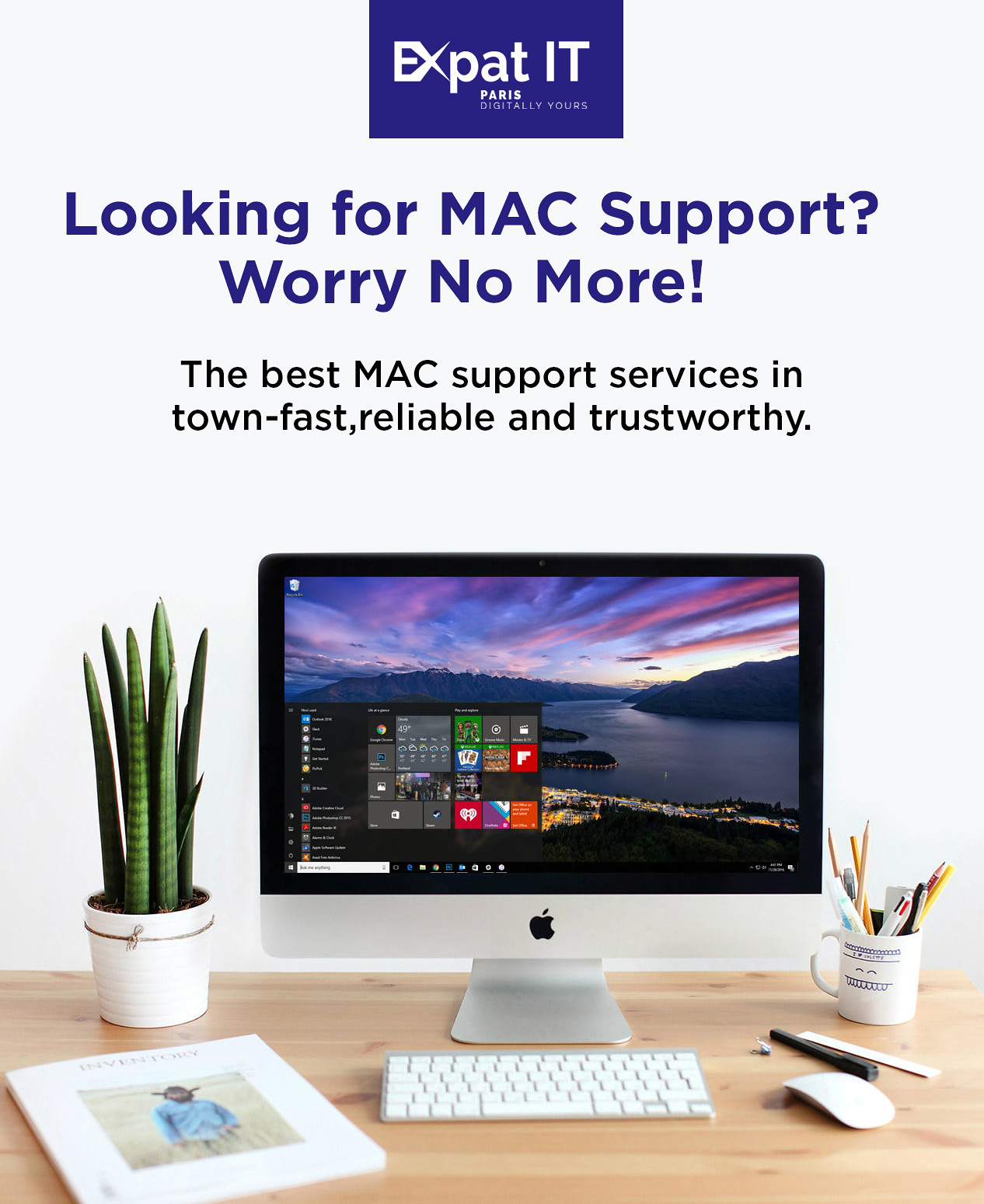The advertisement features prominently at the top in a blue box with white text that reads, "Expat IT Paris, Digitally Yours." Below this, bold blue text states, "Looking for Mac support? Worry no more." This is followed by smaller black text proclaiming, "The best Mac support services in town, fast, reliable, and trustworthy." Showcased in the lower half of the image is a meticulously organized desk setup. At the center stands an Apple desktop computer on a silver base, featuring a distinctive black bezel around the screen. Interestingly, the monitor displays a Windows desktop interface. Surrounding the computer are various items: to the left, a small potted green fern-like plant in a white container and a magazine, while to the right, a white mug filled with pencils and pens. In front of the monitor rests a silver Apple keyboard with white keys, accompanied by an Apple mouse to its right. The overall setup captures a blend of elegance and functional simplicity.